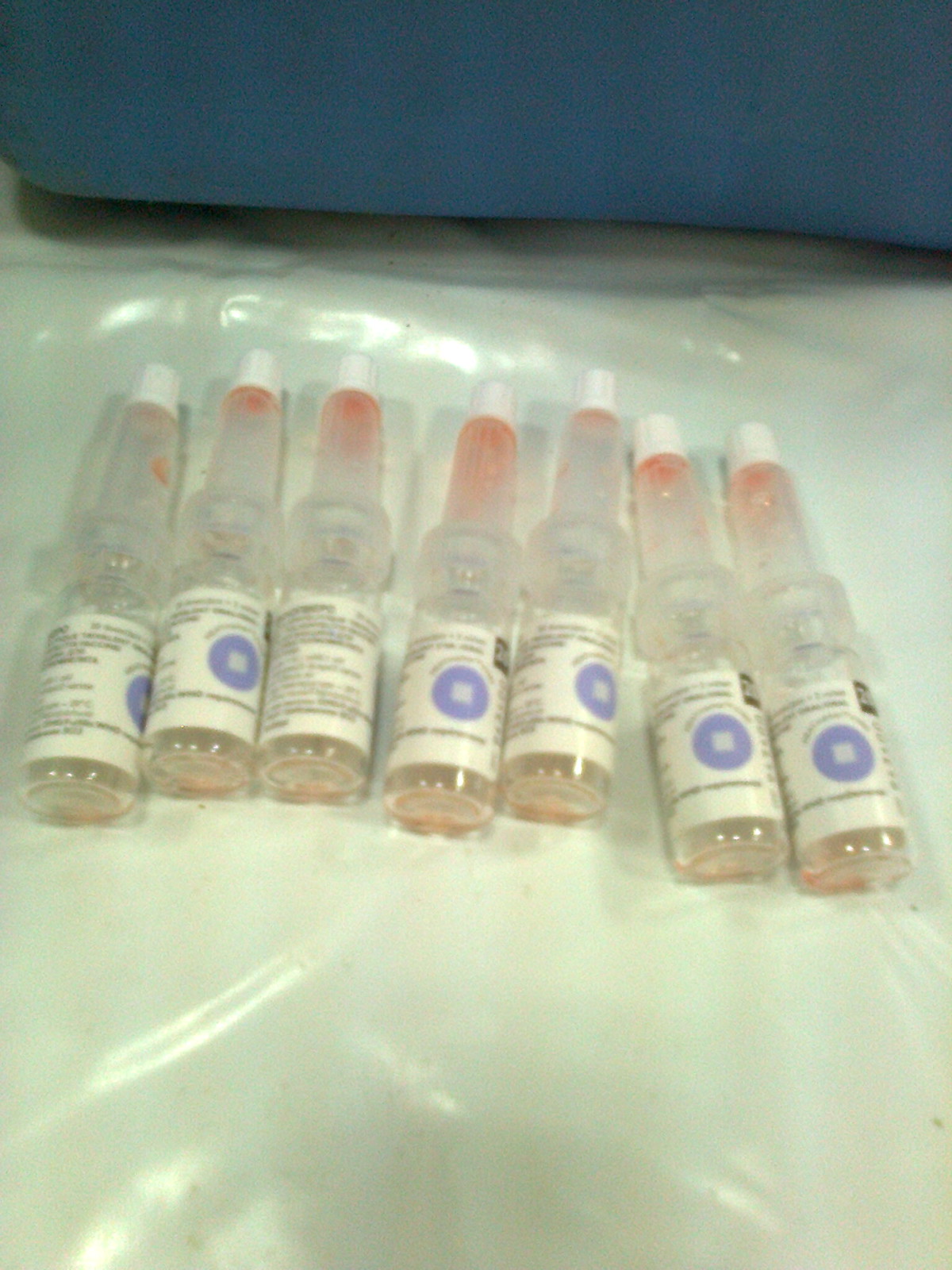This close-up photograph depicts seven elongated, clear glass vials arranged side by side on a white plastic surface. Each vial features a white plastic cap and a white label with small, illegible black text. Prominently displayed on the labels is a blue circle with a white center. A notable characteristic of these vials is the presence of a red staining: the first vial has red liquid near the top, the second near the cap, the third has red towards the middle and top, the fourth has red from the middle upwards, and the fifth through seventh vials show smaller red stains, especially towards the tops. The background of the image is a solid navy blue, possibly part of a chair or sofa, taking up the top portion of the photograph.